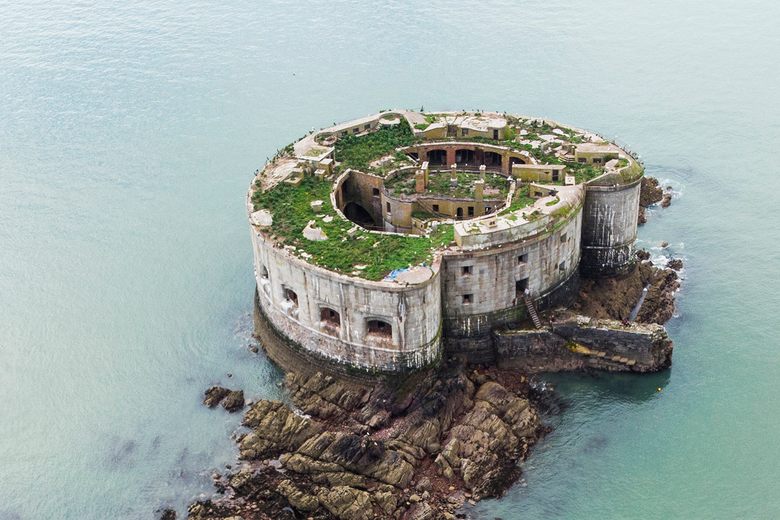The image depicts an aerial view of a weathered, circular stone building situated on a small, rocky island surrounded by clear blue water. The building, likely abandoned, resembles a fort with its cylindrical structure and multiple floors, one of which is partially pushed in. The flat roof of the building is overgrown with green plant life, giving it a partially green appearance. The walls of the building are decaying and exhibit open windows and signs of algae growth at the base. Although very old, the structure remains accessible via a rocky surface connecting it to the surrounding cliffs visible at the bottom of the photo. The scene is bathed in bright sunlight, emphasizing the vibrant blue and teal hues of the clear water. Small figures, possibly tourists, can be seen, one ascending steps leading to the interior of the building.